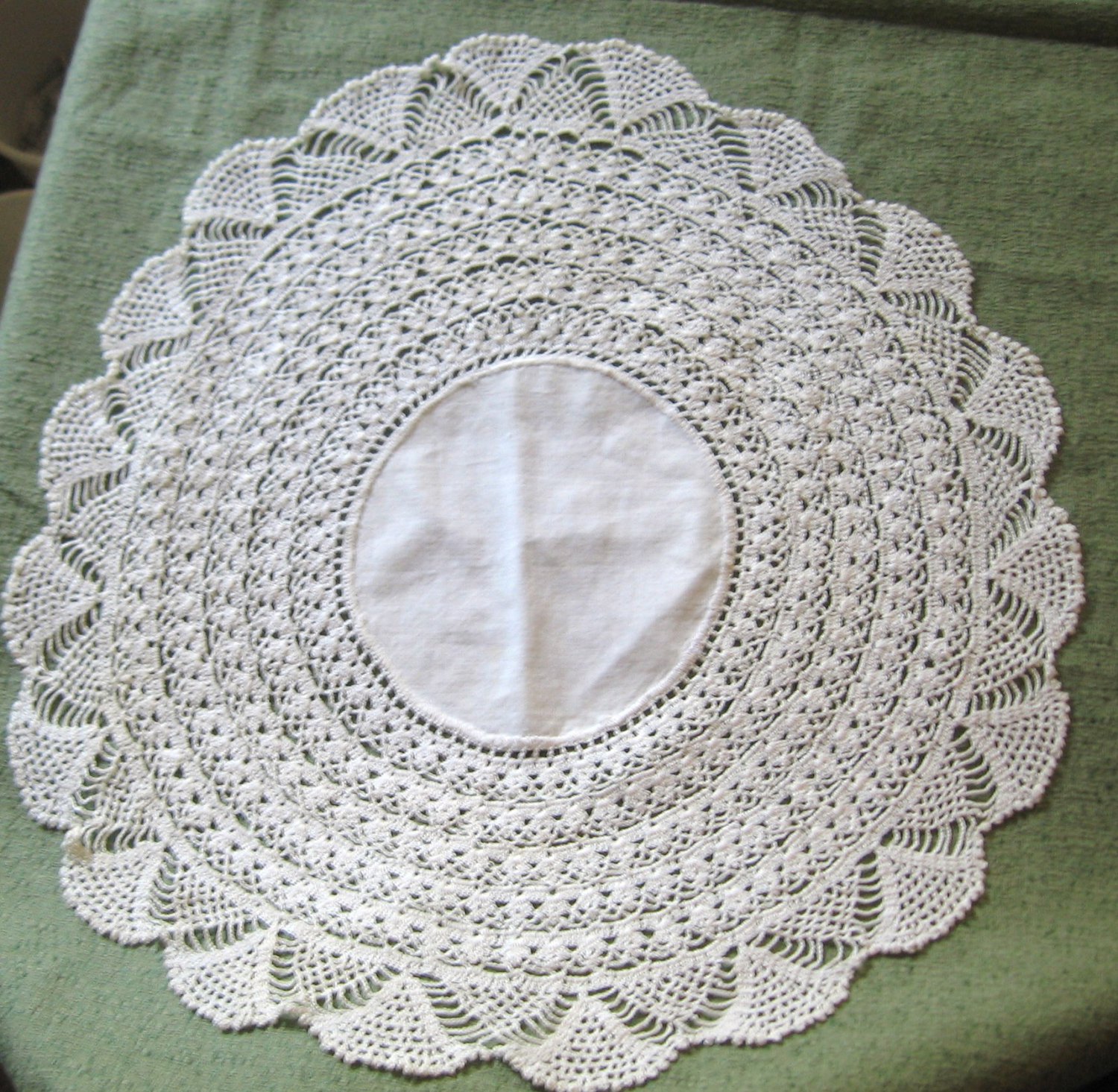The image features a highly detailed, intricately crocheted, white doily resting on a dull greenish-gray fabric background, which appears slightly rough and creased. The circular doily showcases a familiar half-moon pattern along its curvy edges, giving way to about five tighter rows of similar patterns. These designs intricately spiral inward, transitioning from the wavy border into tighter circles until reaching a smooth, solid white center. The doily has a subtle vertical fold line just to the left of its center. In the photograph's top left corner, part of the green fabric extends beyond the doily, revealing a glimpse of what seems to be a plastic container or similar object in the background.